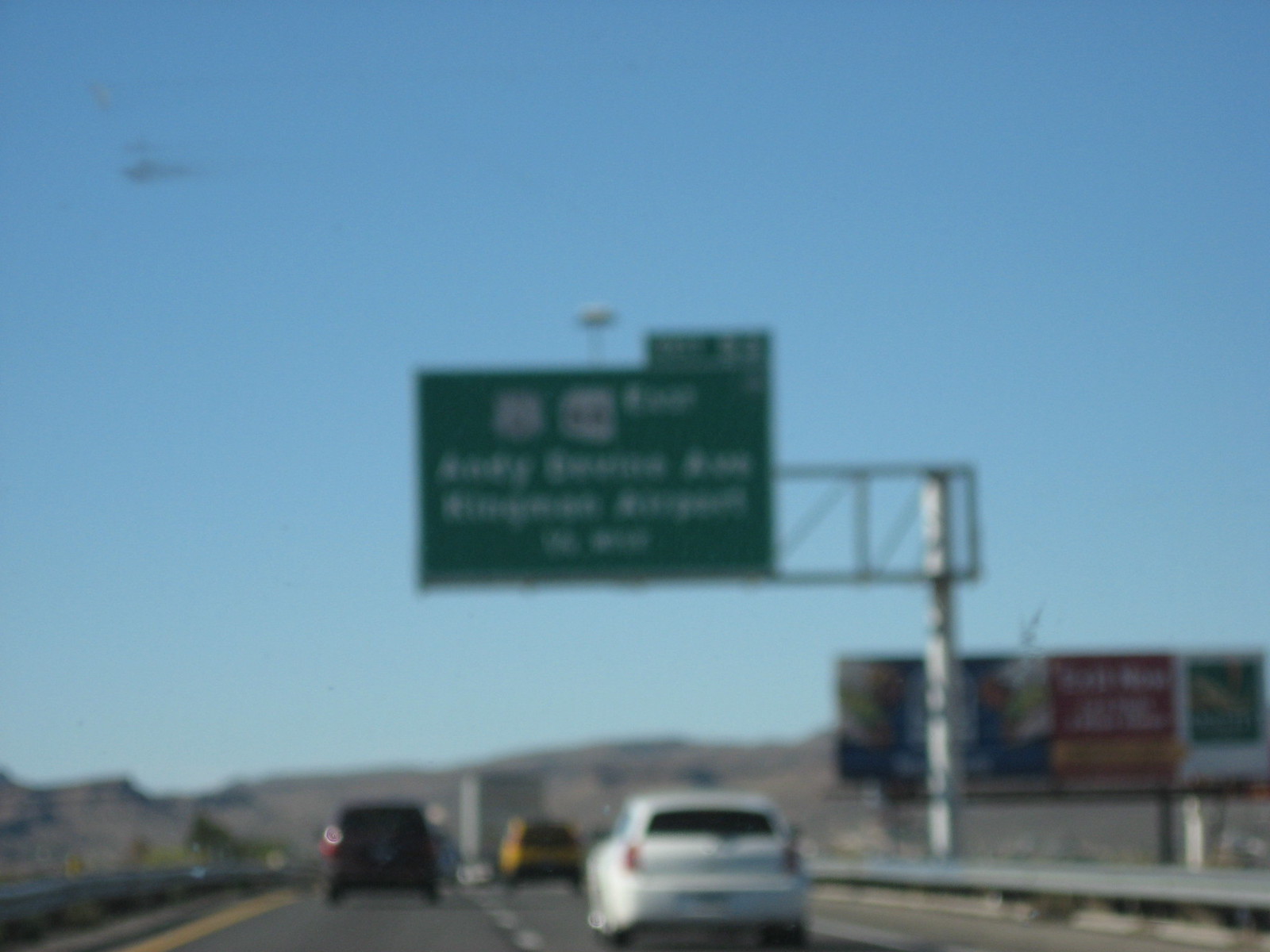The image is a blurry color photo of a highway scene dominated by a bright blue, cloudless sky that occupies the top two-thirds of the frame. In the upper left corner, there's an indistinct object that might be a helicopter. The focal point of the image is a large green road sign with white lettering, unreadable due to the blur, mounted on a stout galvanized metal post extending over the highway. Below the sign, a white car is closest to the camera, followed by a yellow car and a large semi-truck, all traveling away from the viewer. In the left lane, slightly ahead, there is the back of a black vehicle, possibly a van. Guardrails run along both sides of the highway, with two billboards on the right side; one is fully visible while the other is partially obscured. In the distance, the landscape features dry, tree-sparse mountains, possibly placing the location in California or a similar arid region. The photograph appears to have been taken from a vehicle in motion, adding to the overall blur.